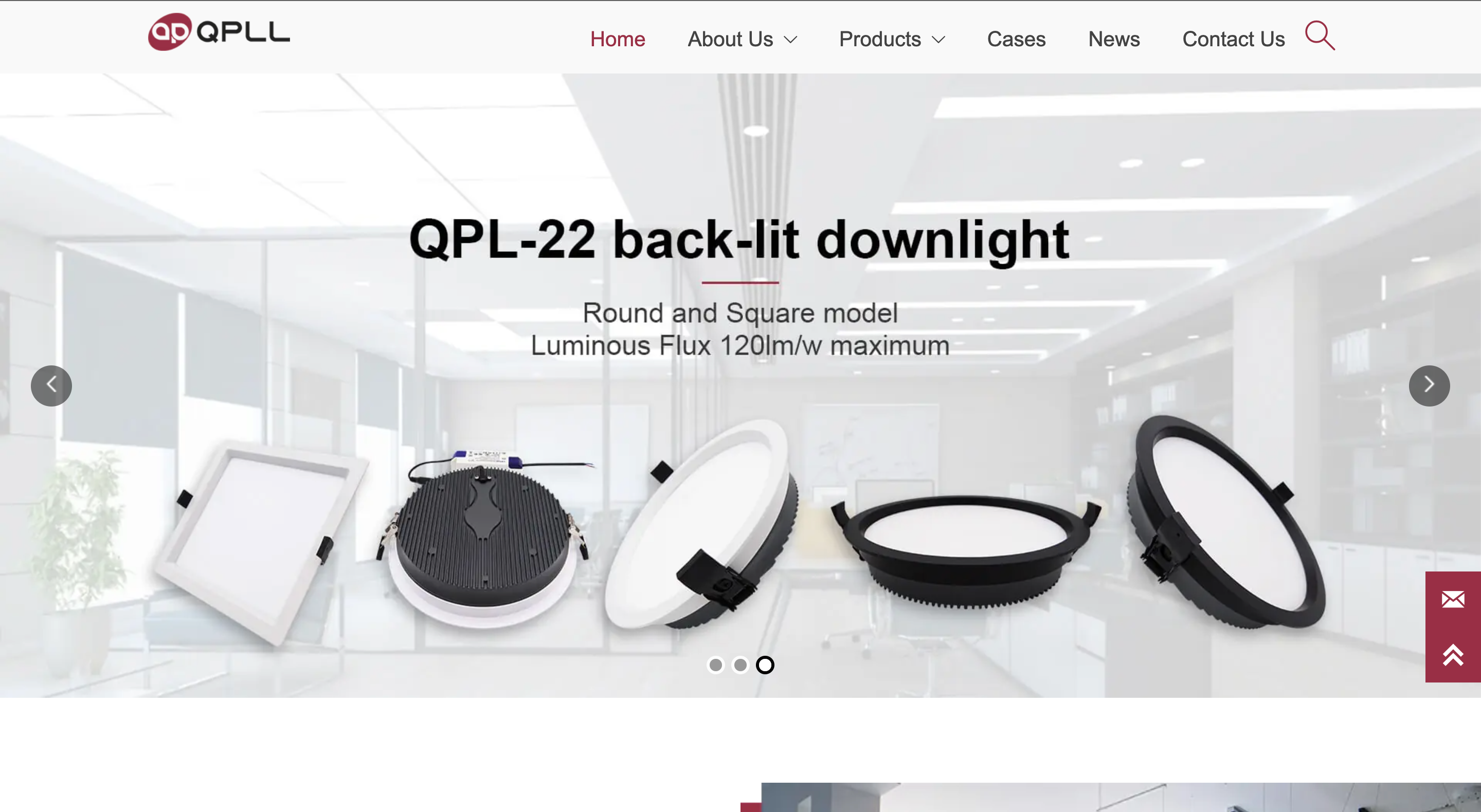A partial screenshot of a website displayed in landscape mode, starting just below the address bar, reveals a user interface with a thin gray banner across the top. On the left side of the banner, the text "QPLL" appears next to a small red logo. To the right, a navigation menu includes options such as "Home" (highlighted in red), "About Us" with a drop-down menu, "Products" with a drop-down menu, "Cases," "News," "Contact Us," and a search function indicated by a magnifying glass icon.

Directly below the menu, there is an image of a simulated office setting, which appears slightly whitewashed. Superimposed on this image in bold text is "QLP-22 Backlit Downlight," with a short red line beneath it. Below the line, in smaller text, are the words "Round and Square Model" followed by "Luxurious flux, 120 [measurement] maximum."

The main content area features five product images of cylindrical or square-shaped objects. Navigation arrows on the far right and left sides of the product display allow users to browse through different pages of products. Below the products, three dots indicate pagination, with the third dot filled in, signifying the current page. A partial image is visible in the bottom right corner, though it is cut off, making it indistinguishable.